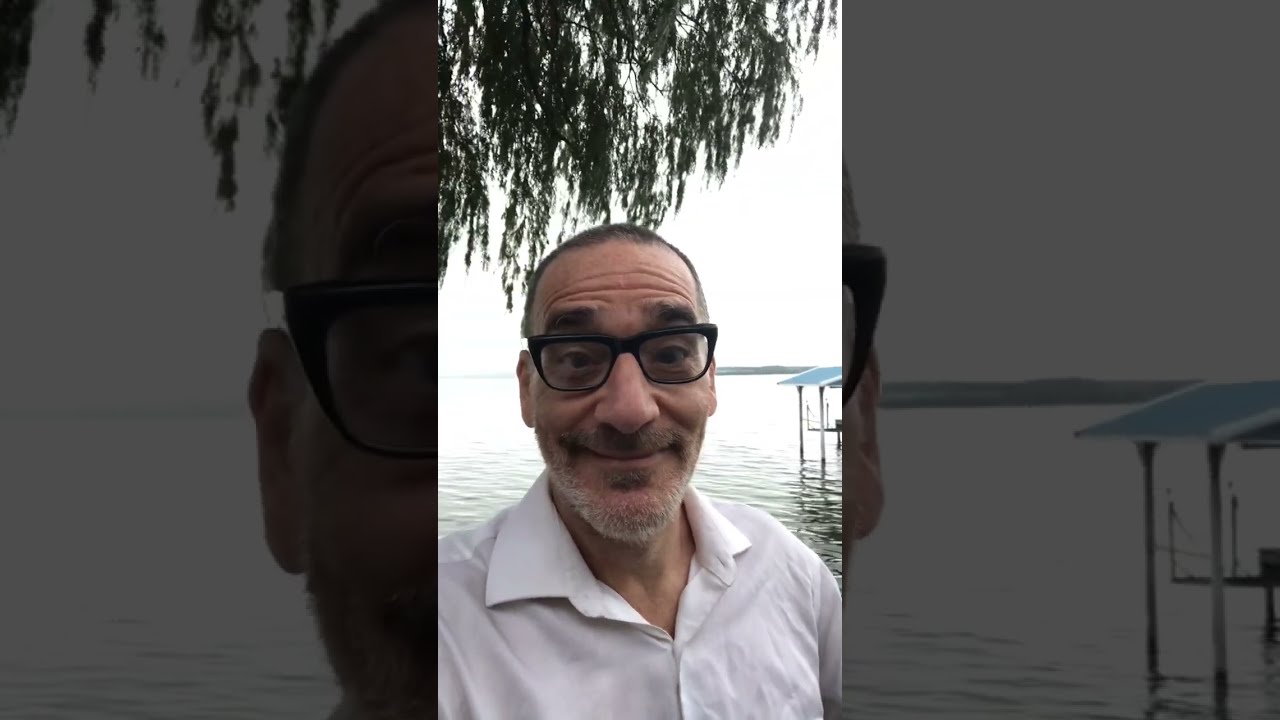This horizontal rectangular image features a man centered between two darker, black-and-white close-ups of his face. The man's primary portrait occupies a vertical rectangle in the middle. He is smiling and looking directly at the camera, wearing black-rimmed, somewhat squarish glasses, and a white collared button-down shirt. His hair is very short and brown, with visible wrinkles on his forehead from his raised eyebrows. His beard and mustache are lightly grown, comprising brown and white strands.

The backdrop showcases a tranquil body of water with gentle ripples, over which a bright white, daytime sky and distant mountains are visible. Some long, green leaves from a tree hang down into the frame, adding a natural element to the composition. There are also some structures like an awning with poles emerging from the water, positioned to the right of the man.

Flanking the central portrait are two vertically wider rectangles. On the left side, the close-up captures about one-fifth of his face, focusing on the eyeglass part, ear, and a hint of his beard, set against a backdrop that includes sprigs of hanging tree leaves and the water. The right side similarly shows only a sliver of his face, mainly the edge of his glasses and ear, emphasizing the water and the structures within it more prominently.

Overall, the image seems to document a serene outdoor setting by a lake, possibly taken as a casual selfie in the middle of the day.